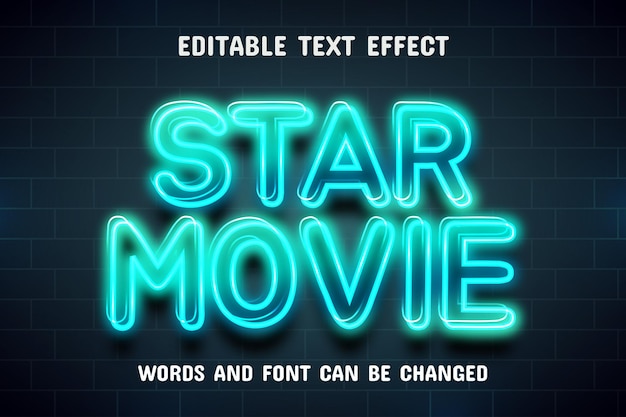The image depicts a graphic design concept with a modern, attractive aesthetic. The background consists of navy or black subway tiles with gray grout, creating a clean and sophisticated backdrop. Prominently displayed at the top are the words "editable text effect" in white. Below that, the phrase "star movie" is presented in a vibrant neon, teal, and turquoise hue, giving it the appearance of a glowing neon sign, some segments outlined in white. Beneath this, more white text reads "words and font can be changed," suggesting that this design is from a text font-changing program, possibly like Canva. Overall, the image showcases an advertisement for a customizable text effect, highlighted by the luminous and eye-catching "star movie" lettering.